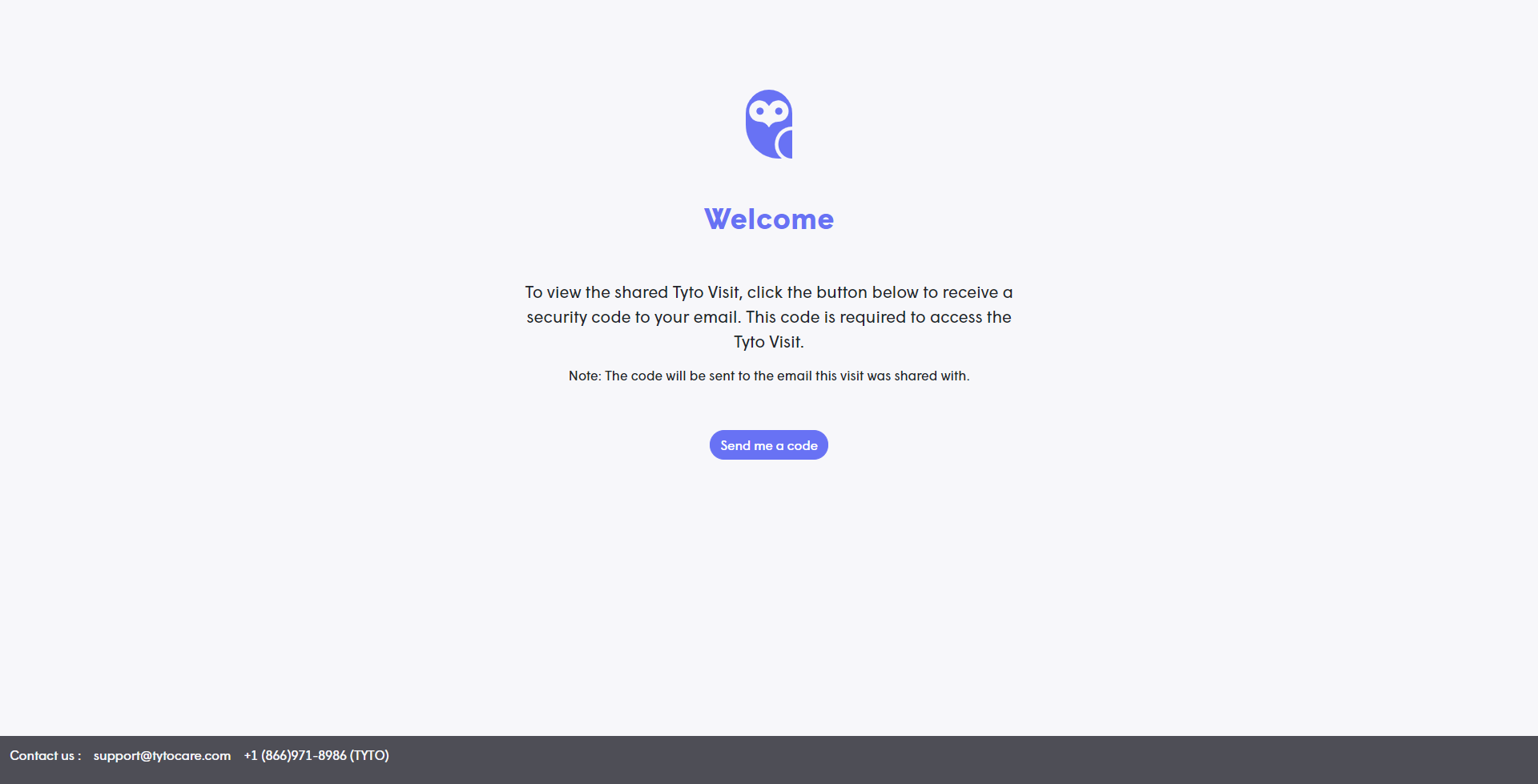The image displays a minimalistic and user-friendly welcome page with a light gray background and predominantly black text. At the top of the page, there is a computer-generated, minimalist illustration of an owl, positioned to appear as if it is looking slightly toward the viewer.

Below the owl, the text welcomes the user and instructs them on how to access a secure section referred to as "tylo visit" (or "tyto visit"). To gain access, the user needs to click a blue button labeled "Send me a code" to receive a security code via email. It is emphasized that the code will be sent to the email address that was used to save this visit.

At the bottom of the page is a black band containing contact information, adding a professional touch to the layout. The overall design suggests this could be related to healthcare or a doctor's visit, where verification of identity is necessary before proceeding. The pleasant simplicity and clear instructions aim to enhance user experience, ensuring that accessing the necessary information is straightforward.